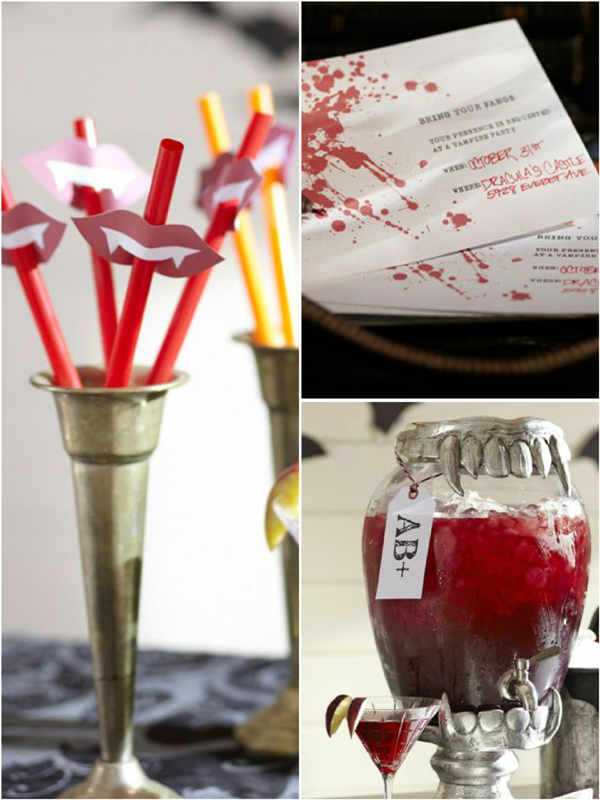The image depicts a detailed arrangement for a vampire-themed Halloween party. Central to the scene is a tall, slender silver or possibly brass vase-like holder containing a selection of red and yellow straws. Each red straw is adorned with paper cutouts shaped like lips, complete with printed white teeth and menacing fangs. The yellow straws are positioned in the background. To the right, a clear glass beverage dispenser is visible, its spout festooned with silver fangs at both the top and bottom. The dispenser is labeled "AB+" alongside a cocktail glass icon, suggesting a blood-themed drink for the event. An invitation is prominently set to the right, stating: "Bring your fangs, your presence is requested at a vampire party on October 31st (Halloween) at Dracula's Castle, 5928 Everett Ave." The decor elements and invitation together convey a meticulously planned, vampire-inspired celebration.